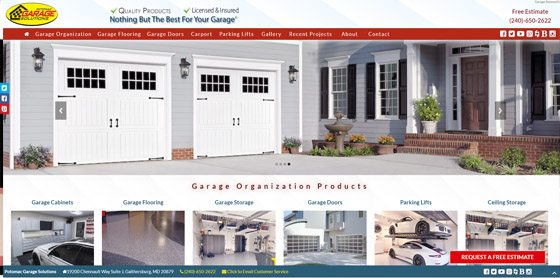The image depicts a professionally designed website for a garage door company named "Garage Solutions." Dominating the top portion of the layout is a banner image showcasing a well-maintained residential property featuring two elegant garage doors, the facade of the house adorned with shutters, flourishing plants, and a charming birdbath. The front door of the house is also visible, adding to the homey aesthetic.

In the upper left-hand corner sits a yellow oval logo that reads "Garage Solutions." Prominently displayed across the top of the image are reassuring slogans and company details: "Quality Products," "Licensed and Insured," and "Nothing but the Best for Your Garage." Additionally, the upper right-hand corner offers potential customers the enticing promise of "Free Estimates," alongside a contact phone number, 240-450-2622.

Central to the page is a section titled "Garage Organization Products," underlining the company's comprehensive offerings. Below this heading are six neatly arranged smaller images representing the different products and services available: "Garage Cabinets," "Garage Flooring," "Garage Storage," "Garage Doors," "Parking Lifts," and "Ceiling Storage."